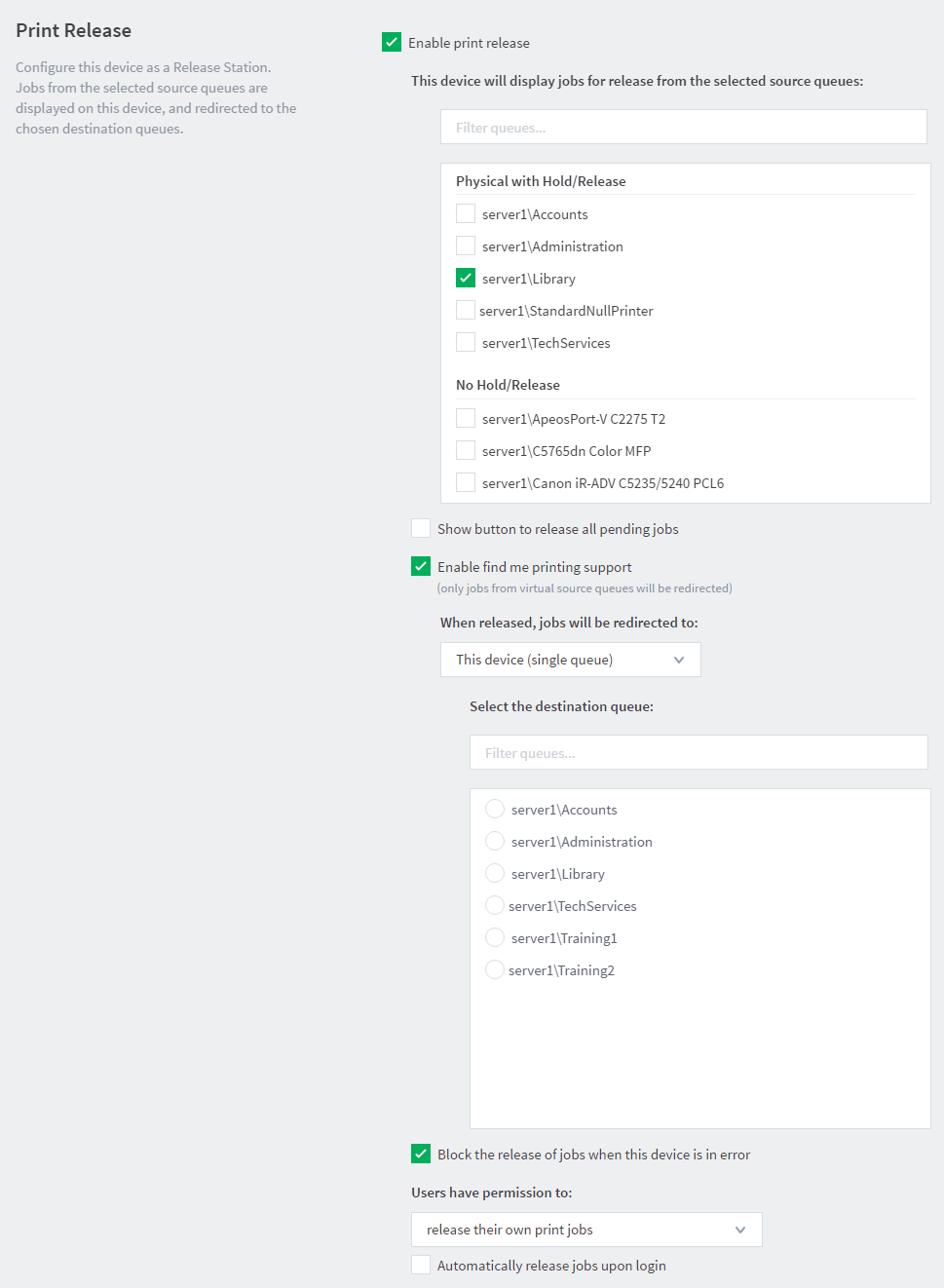**Caption:**

This image showcases the "Print Release" configuration screen for a print management system, wherein a specified device is configured as the release station. The screen contains multiple configuration areas, with several options indicated by checkboxes. Checked options are highlighted in green with a white check mark, signifying they are enabled.

The main areas include:

- **Print Release Enabled:** This setting allows the device to display print jobs for release from the selected source queues.
- **Filters:** Enables various filtering options for print jobs.
- **Physical Withhold Release:** Set to "server1\library," and it is checked.
- **No Hold Release:** Contains three unchecked options.
- **Show Button to Release All Pending Jobs:** This is unchecked.
- **Enable Fine Reprinting Support:** This option is checked.

Below these settings, there are additional indented options pertaining to different user groups such as "server1\ accounts," "server1\ admins," "server1\ library," "tech services," "training1," and "training2."

Additionally, an option to "Block the Release of Jobs When This Device Is in Error" is selected.

At the bottom, the section titled "Users Have Permission To" features a drop-down menu currently set to "Release Their Own Print Jobs."

Overall, the layout is dense with text and checkboxes, indicating various configurable parameters for the print release device.